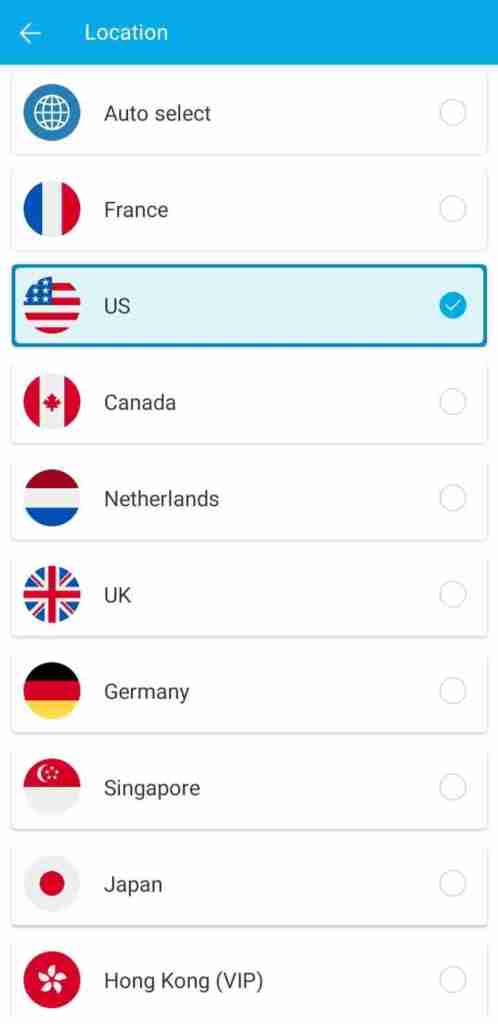The image is a screenshot of a country selection interface. At the very top, a blue header bar displays the word "Location" in white text. On the far left side of this header, a white back arrow is visible. 

Below the header, there is a vertically scrollable list of countries, each divided by a thin line. The countries are displayed with their respective circular flag icons to the left and their names to the right. On the far right, each country has a circular check button.

The list begins with an auto-select option for France. The United States is selected, indicated by a check mark and highlighted in blue. Other available countries include Canada, Netherlands, United Kingdom, Germany, Singapore, Japan, and Hong Kong (noted as VIP). Each country's entry is identically structured with a circular flag icon on the left, the country name in the center, and the check button on the right.